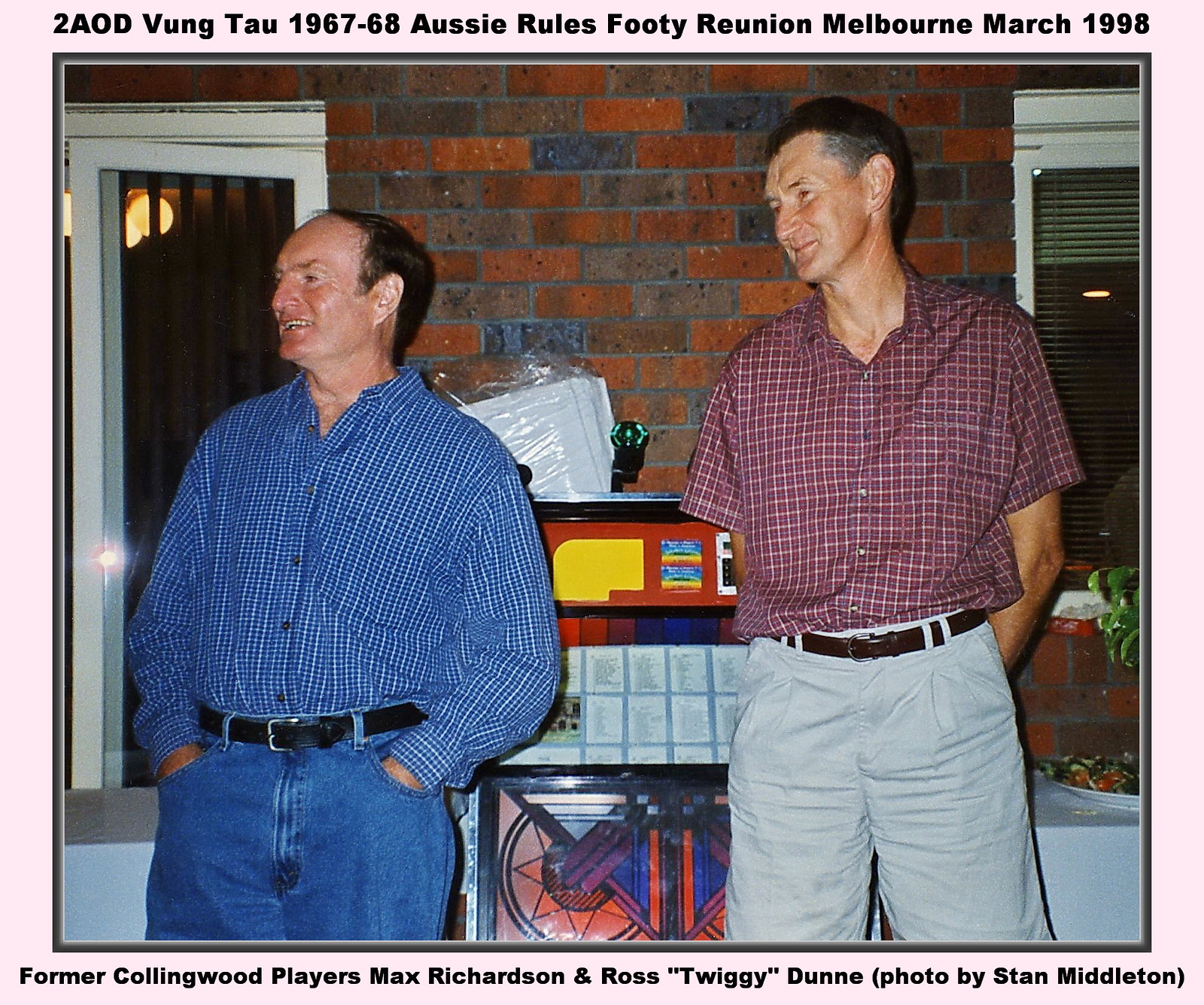In this detailed image, two older gentlemen stand in front of a colorful brick wall, creating a striking backdrop with hues of gray, red, and brown. The gentleman on the left, who is shorter and a bit plumper with a balding head, is dressed in a blue and white button-up shirt featuring a plaid pattern of small squares. He pairs this with blue jeans, a black belt, and has his hands casually tucked into his pockets. The taller and thinner gentleman on the right wears a burgundy-red short-sleeve button-up shirt adorned with thin white plaid lines. He complements his outfit with khaki pants and a brown belt, his hands positioned behind his back, showcasing his full head of hair. Behind them, a window framed in white borders and stained glass, along with rows of text etched above and below, capture attention. At the top, it reads, "T.A.O.D., 1967-68 Aussie Rules Footy Reunion, Melbourne, March 1998." Below the image, the caption identifies the men as "former Collingwood players Max Richardson and Ross 'Twiggy' Dunn," with the photo credit going to Stan Middleton. Additional details in the background include faintly visible boxes or machinery, adding subtle depth to the scene.